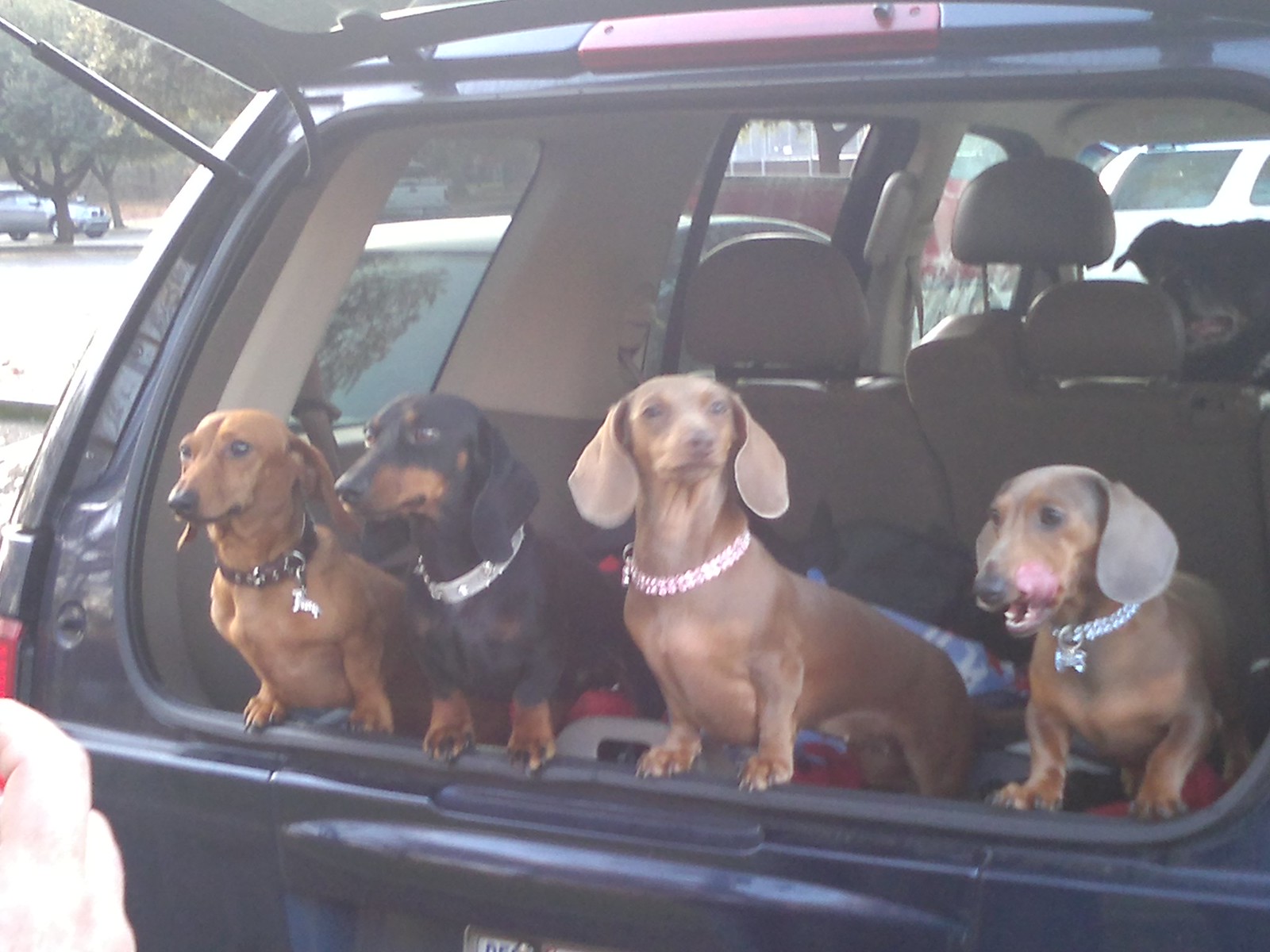In the photo, a family of wiener dogs, or Dachshunds, are positioned in the back of a modern car that resembles a Studebaker or wagon, but isn’t quite an SUV. The hatch of the car is open, revealing a spacious trunk with two rows of seats and possibly the third row folded down. In the background, another larger dog of a different breed, likely a mutt with short ears, is faintly visible. The four Dachshunds, each with distinct coat colors and patterns, are vividly captured. One is a gingery brown, another is black with brown spots resembling a Doberman's markings, a third is a light brown, and the fourth has a mix of light brown and gray tones. They are adorned with fancy collars bearing various charms: one collar is all black, another is bejeweled white, a third is bejeweled pink, and the last has a chain link with a silver dog bone charm. Their heads are poking out of the open hatch, seemingly eager to leap out. The interior of the car appears black with possible red accents, and the blurry image also hints at the presence of fingers in the lower-left corner.